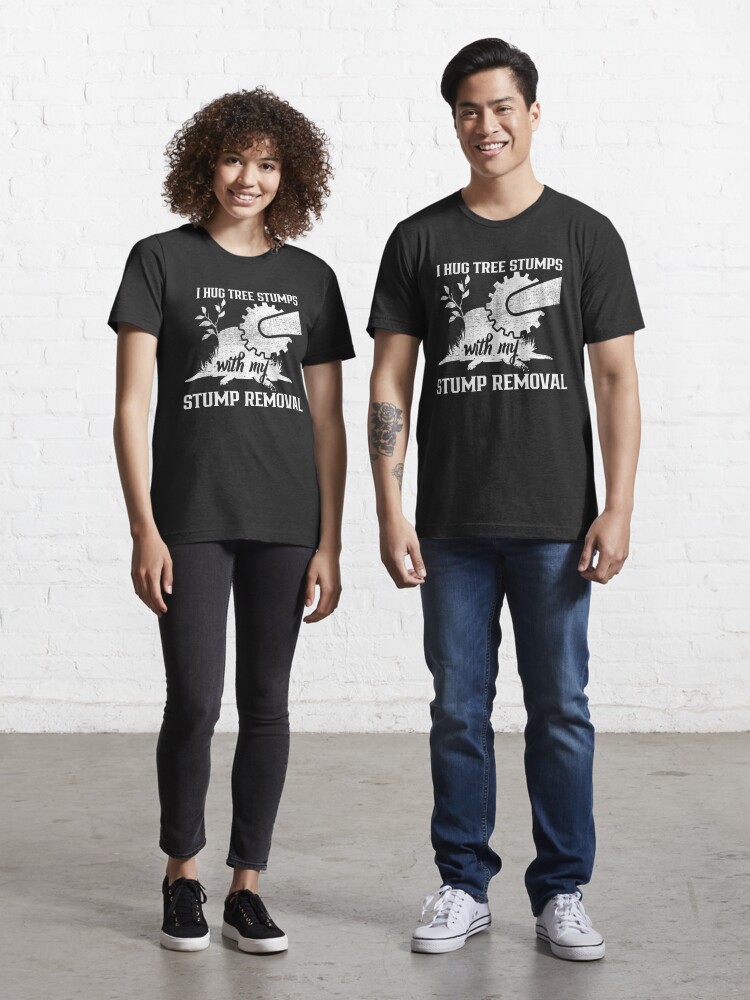In this photo taken inside a studio, a mixed-race woman and an Asian man stand casually in front of a white-painted brick wall and a gray concrete floor. Both are dressed in casual streetwear, sporting identical black t-shirts with a unique design. The t-shirts bear a playful slogan, "I hug tree stumps with my stump removal," accompanied by an illustration of a saw cutting through a tree stump with leaves sprouting from it. The woman stands on the left, her long brown curly hair framing a smiling face, and wears black jeans that are slightly short, black sneakers with white soles, and has disproportionately long arms reaching down to her mid-thigh. The man on the right, with short dark hair and visible arm tattoos, complements her look with blue jeans and white shoes. Both models exude a relaxed vibe, effortlessly highlighting the distinct t-shirt design they are modeling.